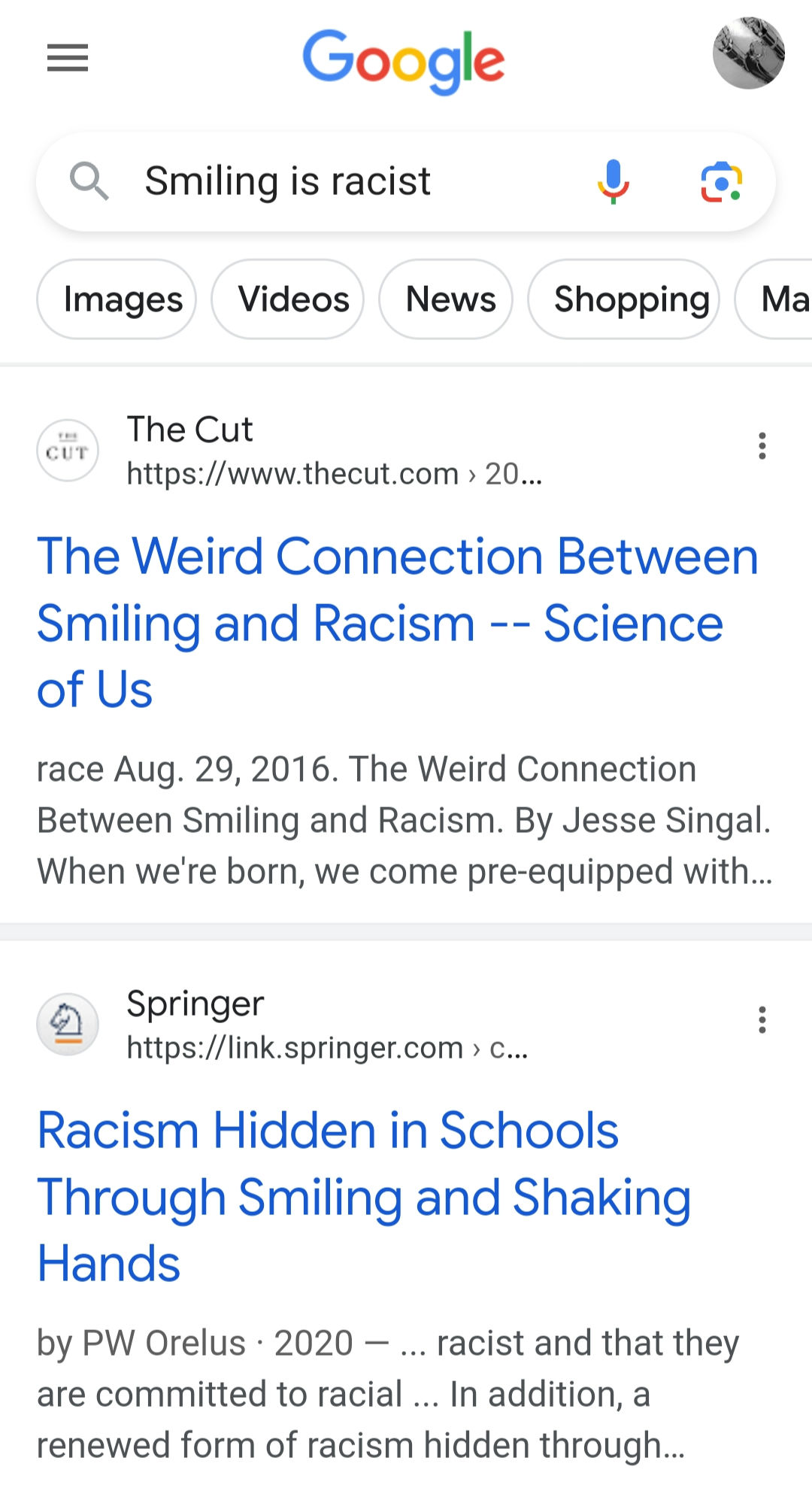A Google search result is displayed in the image. The search query at the top reads, "smiling is racist." The first result is an article titled "The Weird Connection Between Smiling and Racism," authored by Jess Singhal, dated August 29, 2016. The snippet from this article starts with, "When we're born we become pre-equipped with," but the text cuts off there.

The second search result is from Springer, an article by P.W. Orelis published in 2020, titled "Racism Hidden in Schools Through Smiling and Shaking Heads." The snippet for this article mentions, "racist and that they are committed to racial," followed by an ellipsis indicating incomplete information. The text further suggests that more details can be found or additional information can be obtained by contacting the Google search team through their website or the email address provided.